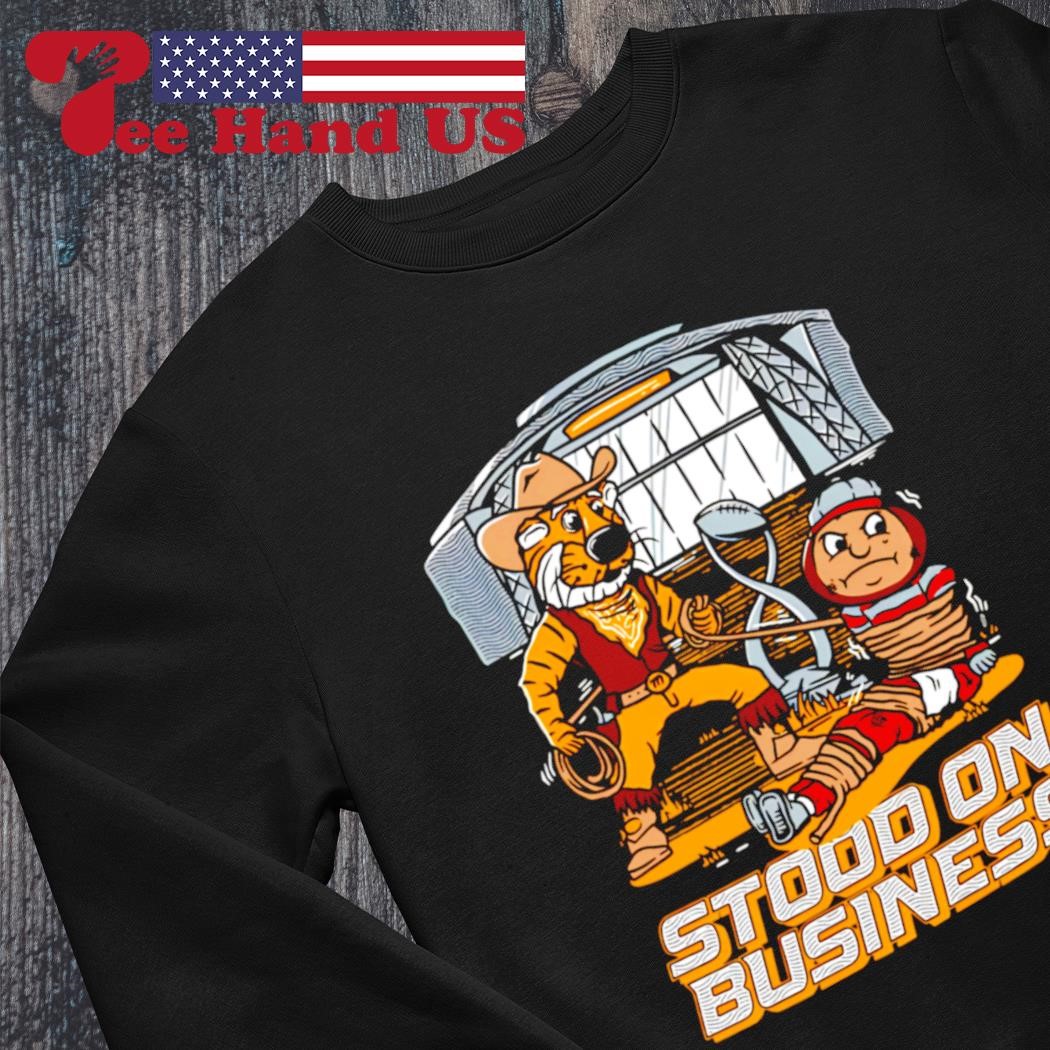In the photo, there's a detailed image of a brand-new black sweatshirt with a crew neck collar. The centerpiece of the design is a vivid illustration of a cowboy tiger, who looks somewhat like Tony the Tiger, with a grinning face, a black nose, and a beige cowboy hat. The tiger is depicted in a full cowboy outfit, complete with an orange handkerchief, a red vest, and boots with fringe. He holds a lasso in one hand, which is used to tie up a frowning character dressed in a red suit with a blue cap. The tied-up figure has a sad and angry expression, with darting eyes, a large nose, and brown eyes, bound tightly around the ankles, thighs, chest, and arms.

Above this scene, in the top left corner, there is a prominent American flag with a blue banner and white stars, alongside red and blue stripes. Near the flag is a red, hand-shaped symbol with the letters "P EE HAND US" written around it. The entire image is set against a backdrop that looks vaguely like bridge work or possibly a stadium, contributing to a dynamic and somewhat ambiguous setting.

Beneath the main illustration, the words "Stood on Business" are prominently displayed in bold white and yellow letters, tying together the thematic elements of the sweatshirt. The garment is laid out on what appears to be a piece of wood, adding a rustic touch to the overall presentation.